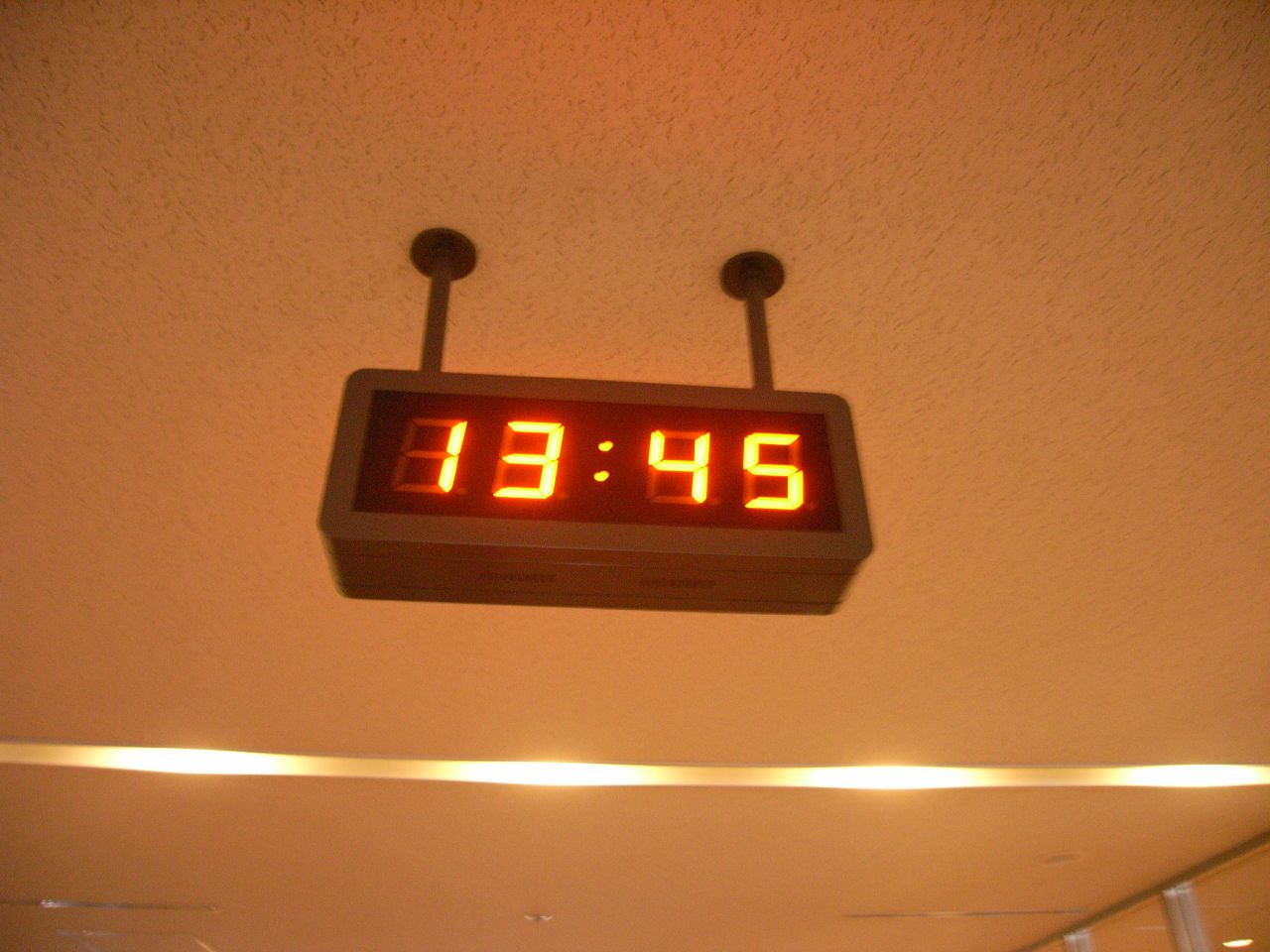In the image, an alarm clock is prominently displayed, suspended from the ceiling and viewed from a low upward angle. The ceiling, a light brownish color, provides a contrasting backdrop. Near the bottom of the image, a white horizontal beam runs parallel to the floor, occupying about 20% of the picture's height. In the bottom right corner, two small gray objects are slightly visible. The centerpiece of the image is the hanging alarm clock, consisting of two black rods and circular fixtures supporting a rectangular frame. The clock itself has a dark outer perimeter, either black or very dark brown, with an inner display that features a black background. The time displayed on the clock is "13:45," with the numbers glowing in an orange hue against the dark display. The rest of the scene is dominated by the ceiling.